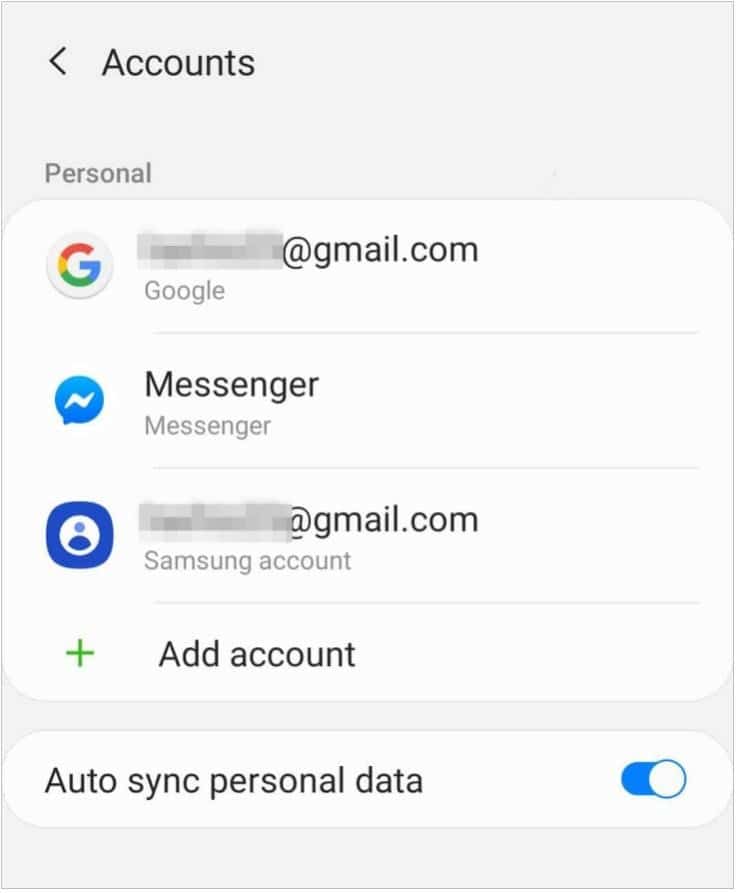This screenshot, taken from an Android or Samsung device, captures the Accounts page. At the top, a left-pointing caret indicates navigation. Below, the word "Accounts" is prominently displayed, with "Personal" in gray text underneath, indicating the personal accounts section. 

The screenshot shows several blurred entries, the most prominent being an email address ending in "@gmail.com," obscured for privacy. Beneath this, three distinct sections appear: 

1. **Google Account**: Denoted by the familiar Google "G," a white circle containing the red, yellow, green, and blue logo.
2. **Messenger Accounts**: Two entries here, each marked by a vibrant blue speech bubble icon with a white horizontal lightning bolt.
3. **Samsung Account**: Represented by a darker blue icon with a white circle containing a blue silhouette of a person's head and shoulders.

Below these entries, a green "Add Account" button invites users to link additional accounts. Additionally, a toggle switch labeled "Auto-sync personal data" is turned on, highlighted in blue.

The background of the page is a light gray, providing a neutral backdrop that makes the various icons and text elements easily distinguishable.